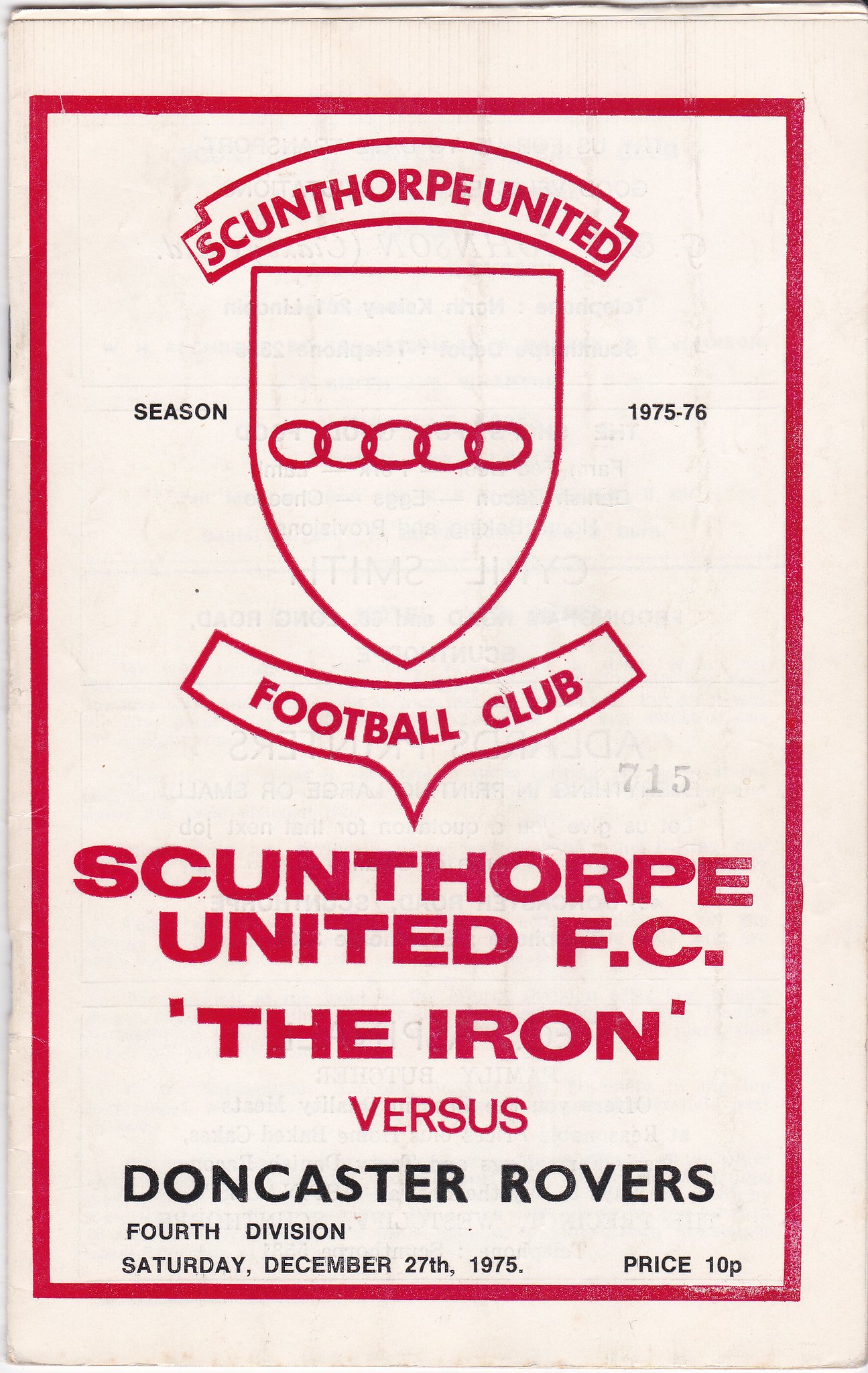This image is a vintage program cover for a football match between Scunthorpe United F.C. and Doncaster Rovers. The background is predominantly light-colored, framed by a narrow red border. Across the top, the text "Scunthorpe United" arches in red. Below this, a red-outlined shield features five interlocked rings in a straight line, resembling Olympic rings. To the left and right of the shield, in black text, it reads "Season 1975-76." Further down, in red text, are the words "Football Club," followed by large, bold letters proclaiming "Scunthorpe United F.C." Underneath, it states "The Iron versus Doncaster Rovers" in smaller red and black text. At the bottom, in black, it specifies "4th Division, Saturday, December 27, 1975. Price 10p."